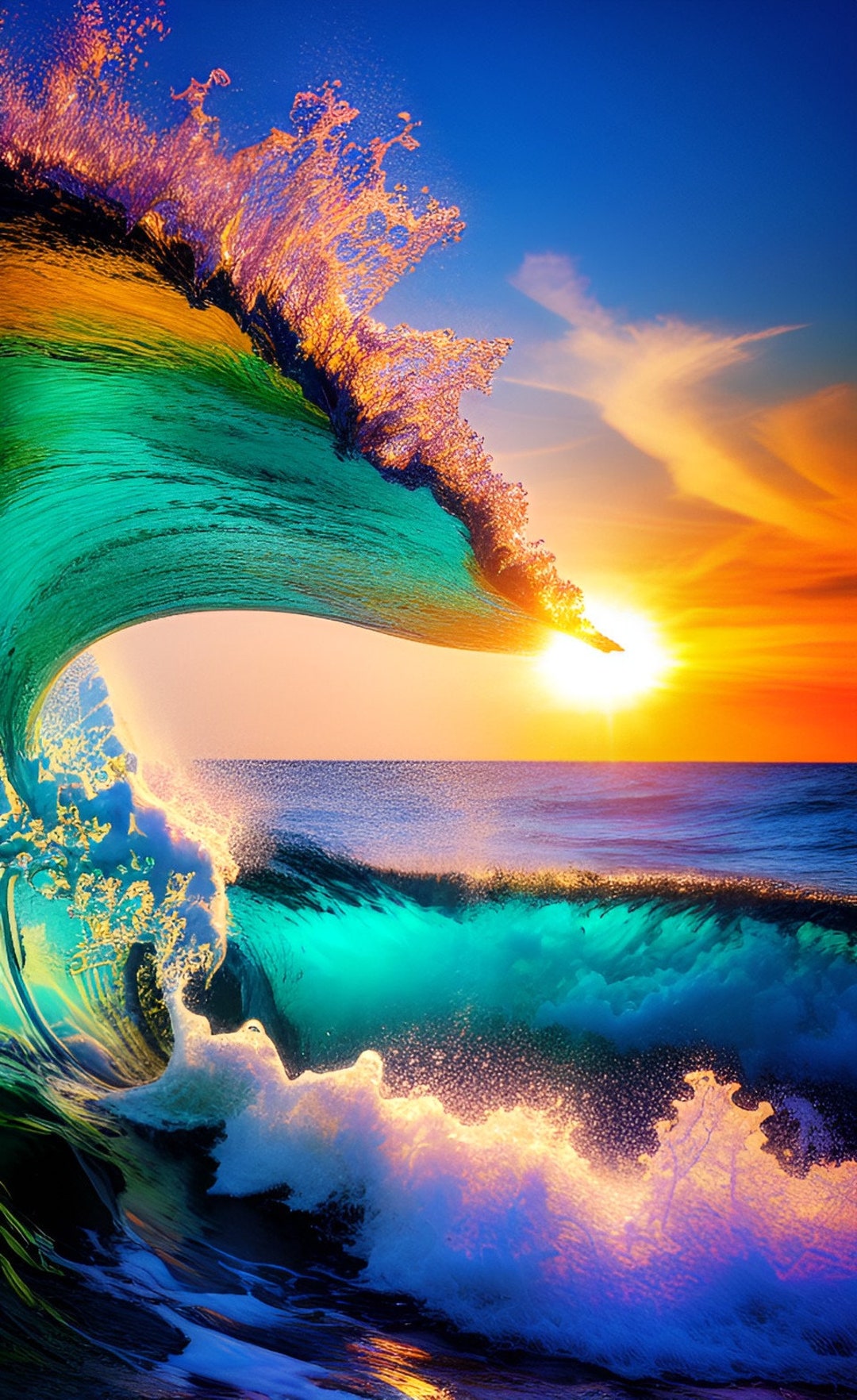The image depicts a highly detailed, computer-generated, photorealistic wave cresting dramatically in the foreground. The wave itself is a vibrant mix of teal, yellow, blue, purple, and green hues, with a dynamic interplay of colors that suggests movement and energy. The cresting wave curls from the top left quadrant into the center of the frame, with foam and white bubbles indicating active turbulence in the water. In the background, a vivid yellow and white sun is setting, casting an orange glow across the horizon and blending seamlessly into the royal blue sky. This entire scene is captured in portrait orientation, highlighting the height and perfect surfing conditions of the towering wave, even though no surfers are present. The overall impression is of a stunningly vivid, surreal seascape that combines natural elements with artistic enhancements.